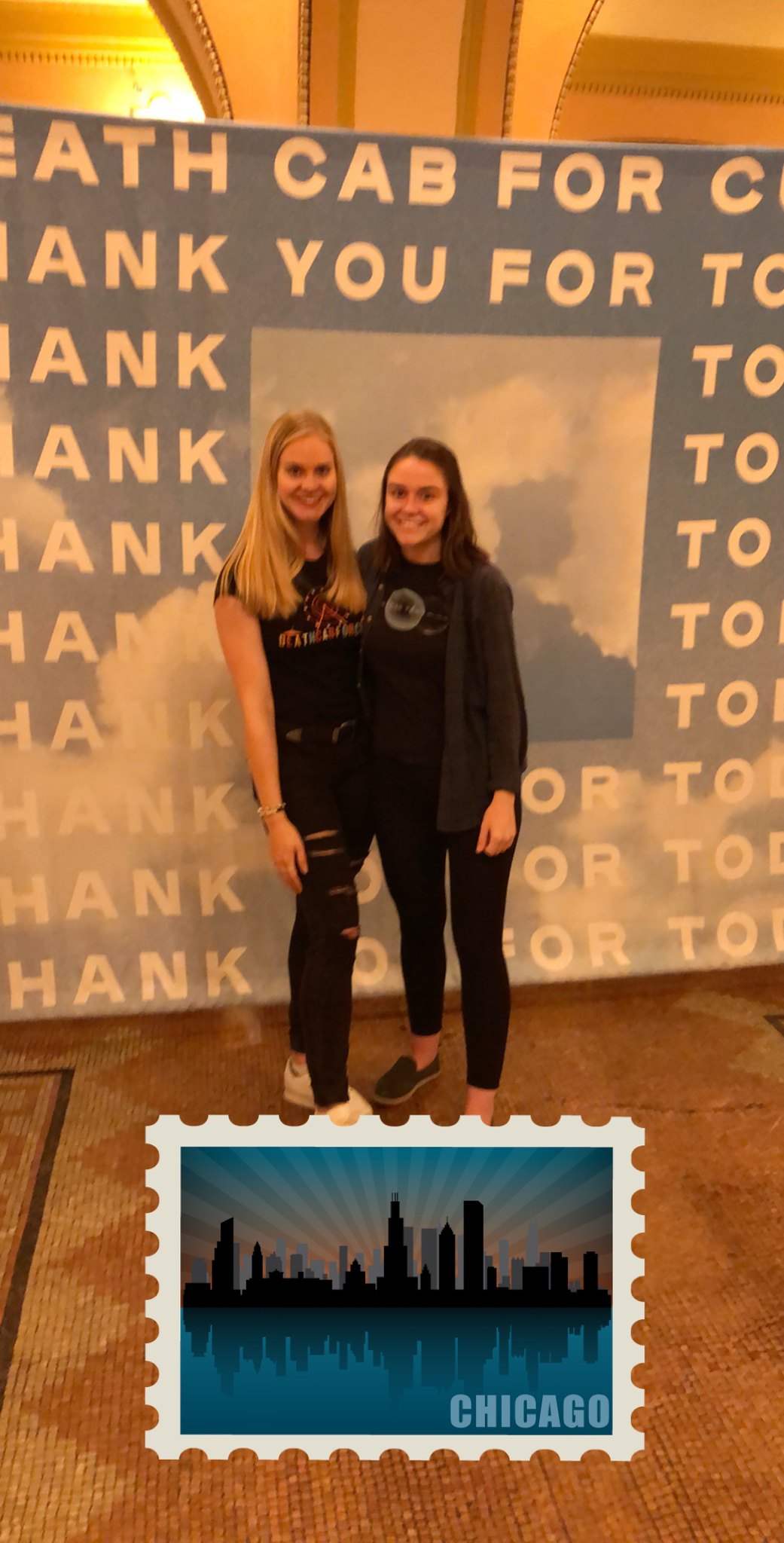In this detailed photograph, two young women stand side by side on a brown tiled floor in front of a sizable sign. The sign features gray at the top with light orange letters, partially spelling out "E-A-T-H" alongside fragments of other words, possibly forming the phrase "thank you for." Both women are dressed in predominantly black outfits: the girl on the left, a blonde, wears a short-sleeved black shirt, black pants, and sneakers, while the brunette girl on the right is clad in a gray sweater over a black shirt, black pants, and black shoes. The scene is further adorned with a poster in front of them, resembling a postage stamp that showcases the blue expanse of Lake Michigan and an outlined drawing of Chicago's skyscrapers. The word "Chicago" is prominently marked in the lower right corner of the stamp. The women, appearing to be between 15 and 18 years old, are positioned against this urban-themed backdrop, creating a striking and cohesive visual.